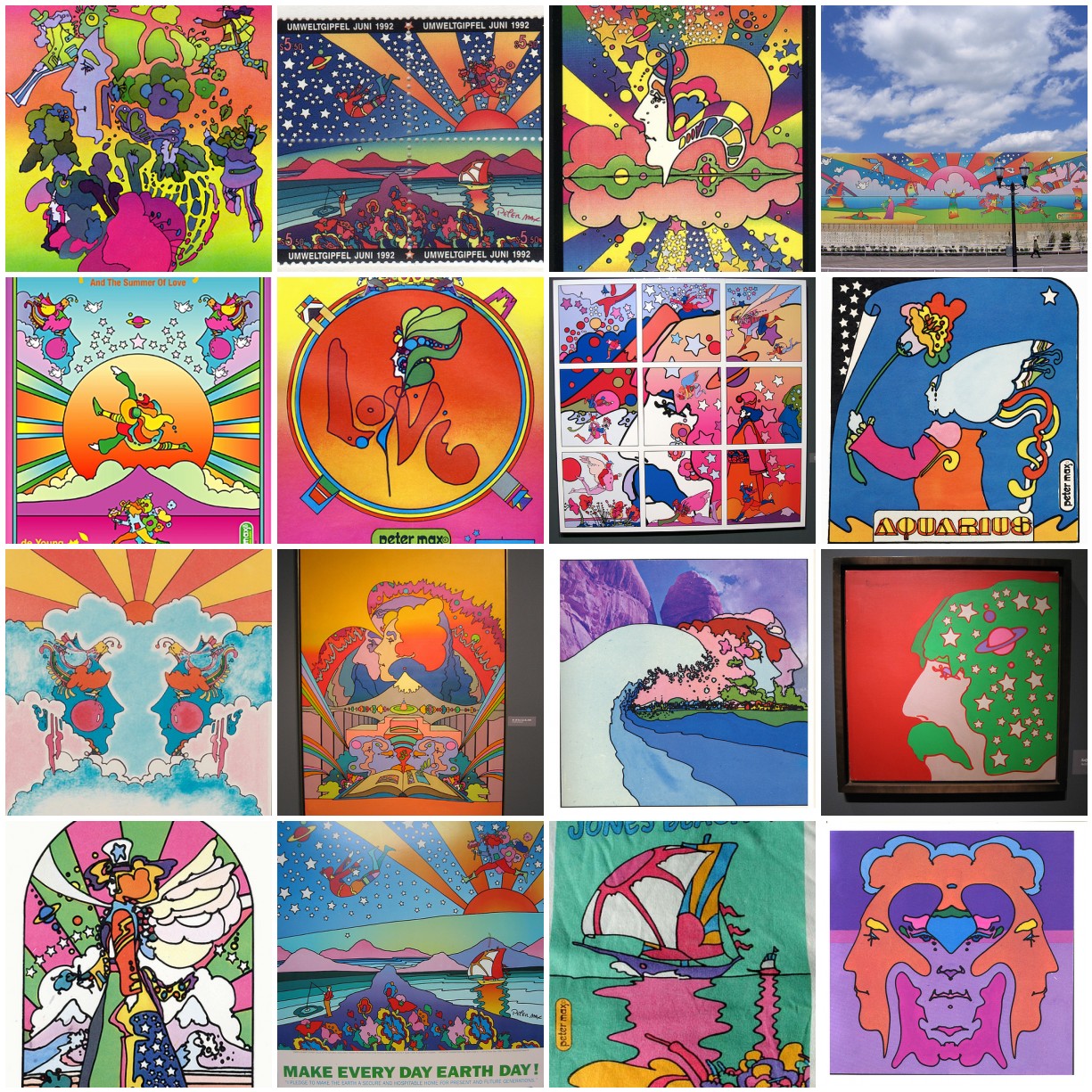The image is a vibrant mosaic of 16 square stickers or artworks, each featuring colorful and psychedelic designs. The predominant theme across these stickers is cartoonish and abstract faces, with one notable illustration of a man's face adorned with a green mustache and green hair filled with stars and the planet Saturn. There’s also a distinct photo of a mural showing a blue sky with white clouds, a recurring motif of nature, sea, and celestial elements. Some stickers contain inspiring text such as "love" in the center of a circle and "make every day Earth Day." The artwork uses a rich palette including red, pink, green, yellow, purple, and gray, contributing to the lively and eclectic aesthetic.